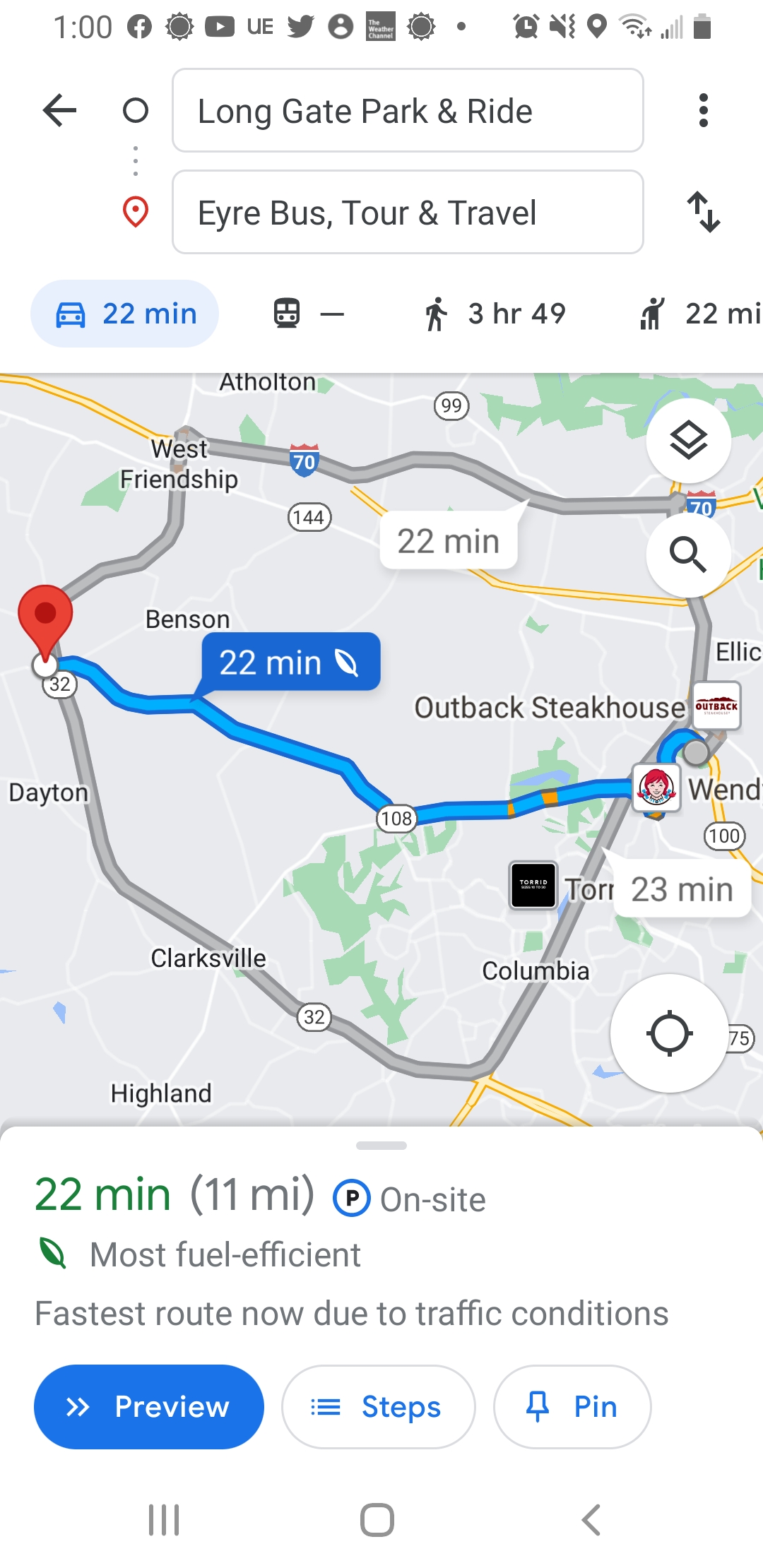This is a detailed screenshot from a smartphone displaying directions on Google Maps. The map outlines a journey of 11 miles, estimated to take 22 minutes by car and 3 hours 49 minutes on foot, from Long Gate Park and Ride to Ayer Bus Tour and Travel. The route prominently features a number of towns including Columbia, Clarksville, Dayton, Benson, Friendship, and Highland. Landmarks along the way include a Wendy's and an Outback Steakhouse, suggesting the route either begins or ends near these locations. The final destination appears to be close to Highway 32. Notably, the map indicates that this is the most fuel-efficient and fastest route available at the current traffic conditions. The timestamp on the image shows it was taken at 1:00 PM, with several apps visible on the phone’s interface.